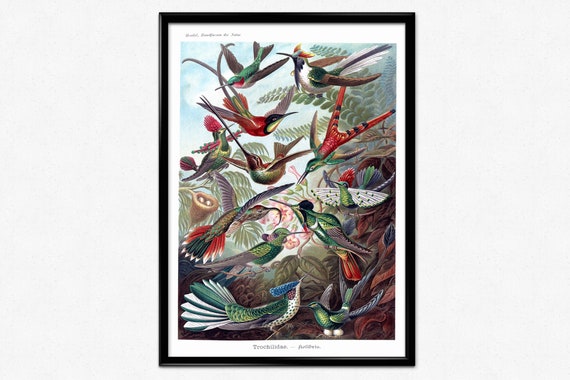The framed image is a detailed painting of various birds, presented in a black frame with a white border. The painting depicts numerous birds, including hummingbirds, all flying or perched amidst lush vegetation. The sky in the background is blue with patches of clouds. The vegetation features diverse species of leaves, primarily green, but some are tinged red at the bottom. Among the birds, there's a striking one with a fanned tail resembling a peacock, sporting a speckled body and blue head. To its right, a bird with a green body and blue wings is seen, and nearby, a bird with white wings and a green body. Another noticeable bird has an olive-colored body and a brown head, while a red-bodied bird is positioned above it. In the upper corners, there are birds with distinctive features: one green with gray wings on the left, and a black-and-white bird with a long beak on the right. Surrounding the birds are large fern leaves, adding to the intricate natural setting. The painting includes unreadable text in black font at the top left and bottom. The artwork, rendered in a style resembling oil or watercolors, captures the vividness and diversity of the avian world.